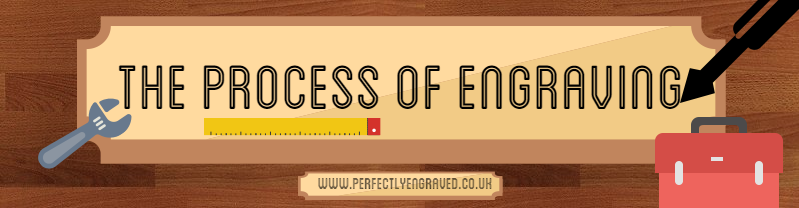The advertisement is a long, thin rectangle with a background of natural wooden slats, showcasing the detailed grain of the wood. In the center of the ad, there's a prominently bordered banner with a light brown edge and a yellowish-beige interior. The banner contains the phrase "The process of engraving" in bold black font. Extending from the lower right corner of the final "G" in "engraving" is an illustrative arrow-like engraving tool, pointing downward. A small wrench is positioned near the "T" in "the," and a yellow ruler is placed just beneath the word "process." On the lower right side of the ad, there's a red toolbox with a black handle and white buckles. At the very bottom of the ad, another small banner displays the website "www.perfectlyengraved.com.uh" in matching black font on the same yellowish-beige background. The overall composition suggests a promotional piece for a website dedicated to engraving, reminiscent of instructional content.